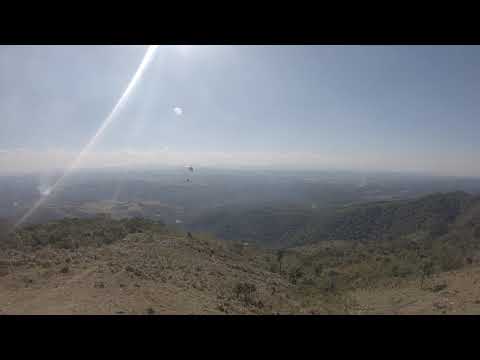This photograph, taken from a mountaintop or hilltop, captures a sweeping valley landscape shrouded in fog or smog, creating a blurred effect across the entire scene. The valley below is predominantly covered in lush green grass and trees, interspersed with occasional brown and tan patches of dirt, indicative of bare patches of land. The foreground closer to the mountaintop appears drier, exhibiting more brown hues with scattered green areas. The sky overhead is predominantly gray, with only distant clouds visible on the far horizon. Sunbeams and reflections suggest the presence of the sun just outside the upper boundary of the image, although the sun itself is not visible. Framed by black horizontal strips at the top and bottom, this atmospheric and detailed image presents a serene, natural landscape with muted colors and a sense of depth.